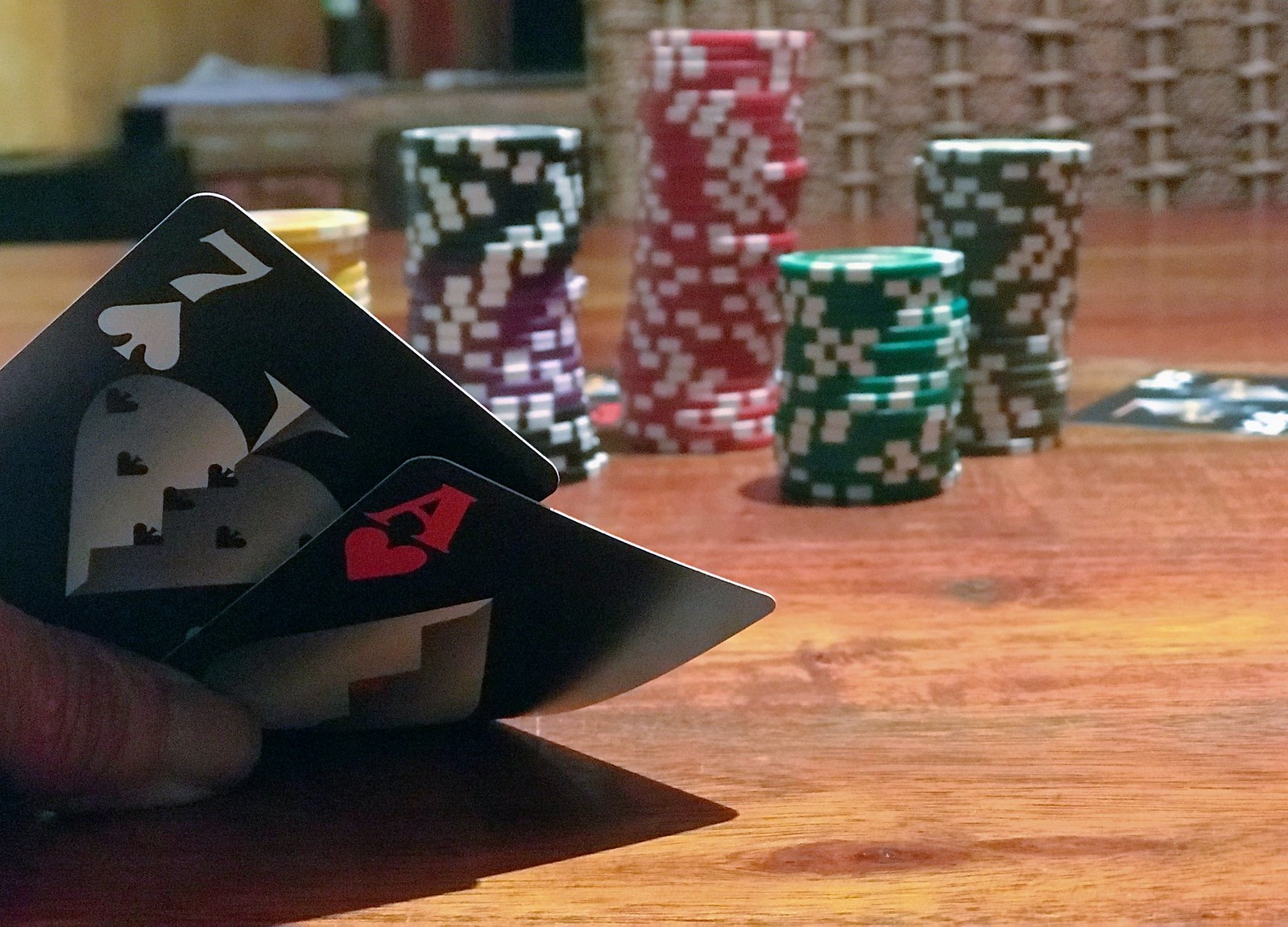The image captures a close-up view of a poker scene set on a brown wooden table. Prominently displayed are five neatly arranged stacks of casino chips, each stack featuring alternating colors of yellow and white, purple and white, red and white, green and white, and a slightly different shade of green and white. In the foreground, a Caucasian hand holds two playing cards: the seven of spades and the ace of hearts, both rendered in black and white with light gray accents. In the background, there is a stack of indistinct objects, possibly the back of a chair, adding depth to the scene.